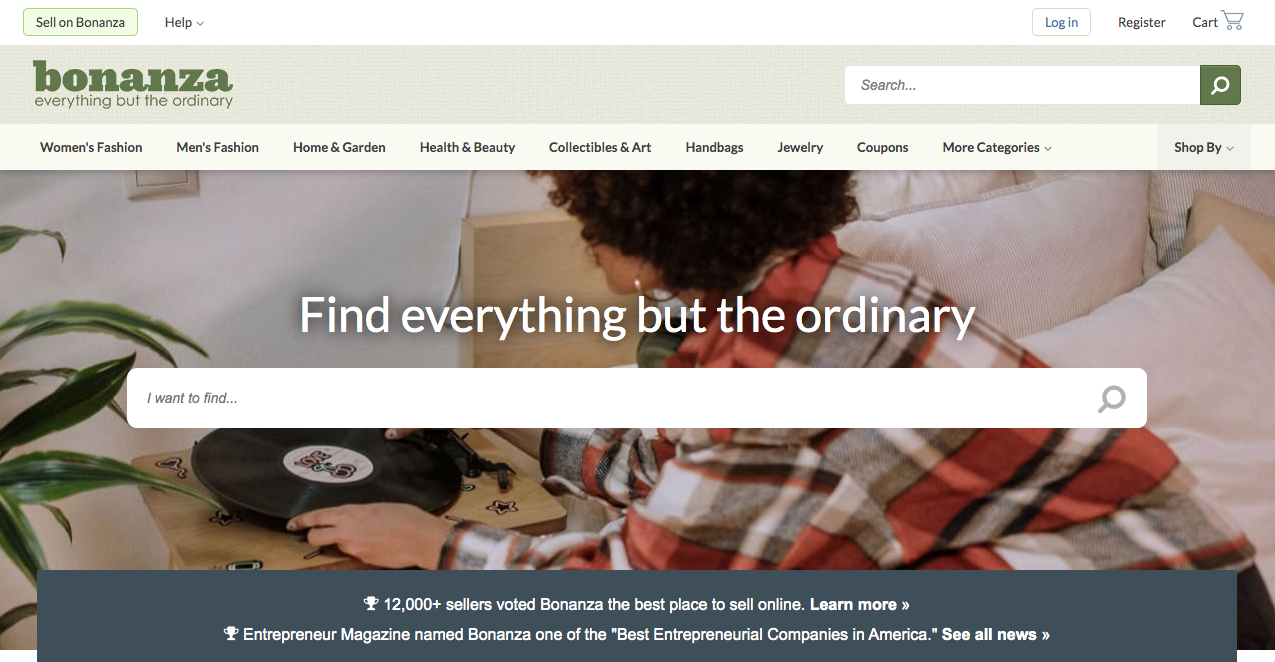Here's a cleaned-up and detailed descriptive caption for the image:

---

The image is a landscape-oriented screenshot of a webpage from the online marketplace Bonanza, viewed on a laptop. The screenshot is roughly twice as long as it is tall and lacks defined borders. At the top of the webpage, there's a narrow rectangular white section containing a green square to the left with black text that reads "Sell on Bonanza." Beside this is a help drop-down menu.

On the right side, there is a thin gray rectangular box with the word "Login" in a distinct BooFont typeface, followed by "'Register" in black font, next to a tiny cart icon. Below this header is a banner with a brownish-green background that prominently displays the word "Bonanza" in lowercase dark Korean letters, alongside the tagline "everything but the ordinary." To the right of this is a white search bar with a green square housing a white magnifying glass icon.

Beneath this banner is another thin white border featuring several subcategory links, including "Women's Fashion," "Men's Fashion," "Home and Garden," "Health and Beauty," "Collectibles and Art," "Handbags," "Jewelry," "Coupons," and additional categories.

A larger image below this section showcases a woman with long, thick curly hair wearing a flannel shirt. She is placing a record onto a record player. Superimposed in the center of this image is a search bar with the prompt "I want to find..." allowing users to input search terms.

At the bottom of the screenshot, within a blue border, a testimonial boasts "12,000 plus sellers rated Bonanza the best place to sell online," highlighting customer satisfaction.

---